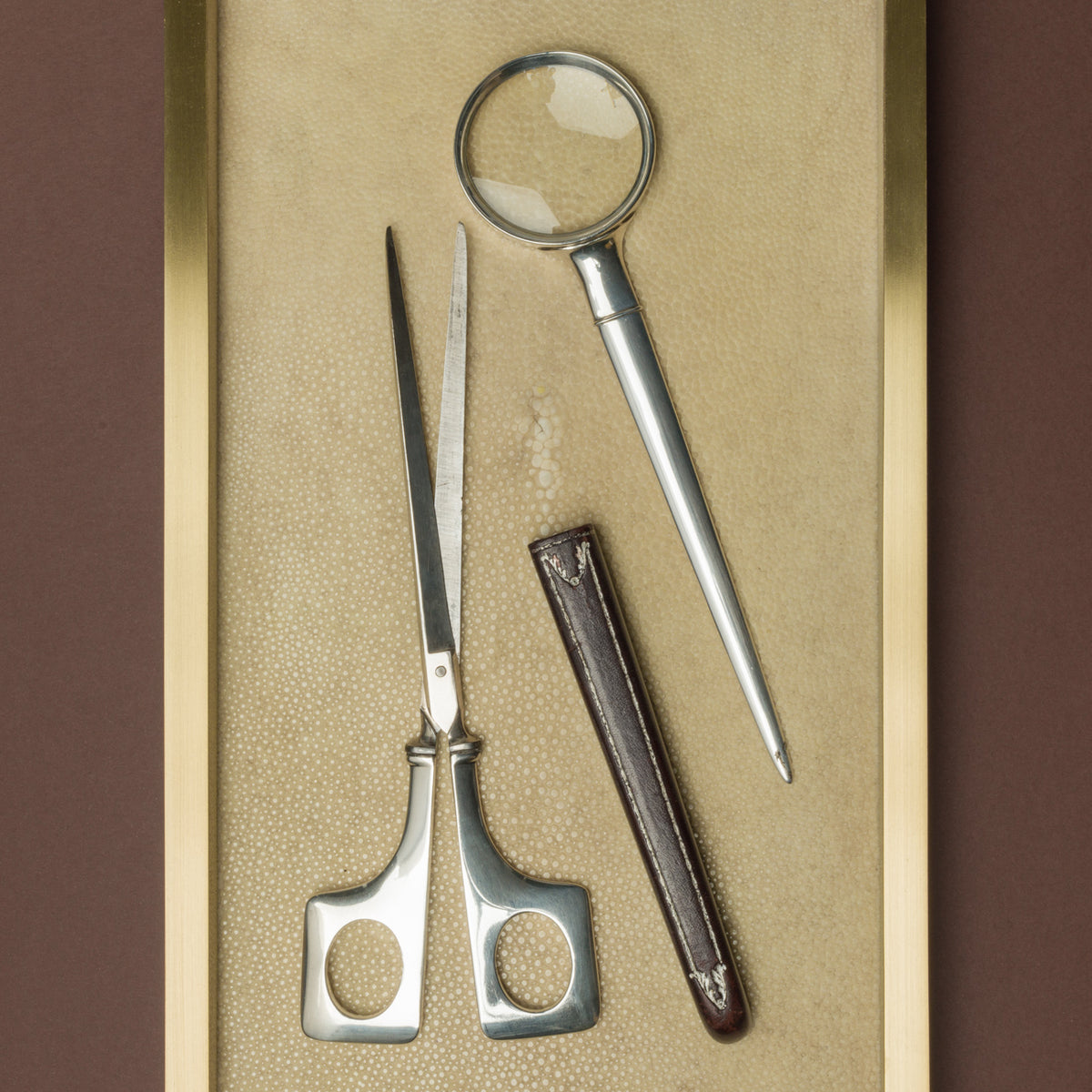Against a dark, maroonish brown background, a brass tray with shiny, metallic borders on either side showcases three intriguing items. The tray appears to have a textured, possibly marbled glass surface. Positioned on this tray are a magnifying glass, a pair of elongated scissors, and a brown leather scabbard. The magnifying glass, with its silver outline and pointed end resembling a letter opener, lies at the top right, extending upwards. Below and to the left of the magnifying glass are the scissors, featuring distinct, squared-off handles for finger placement, and laying upside down with the handles at the bottom of the image. The brown leather scabbard, situated between the magnifying glass and the scissors, looks like it could house either tool. Both the magnifying glass and the scissors have a metallic, stainless steel finish, adding to the antique aesthetic of this detailed composition.